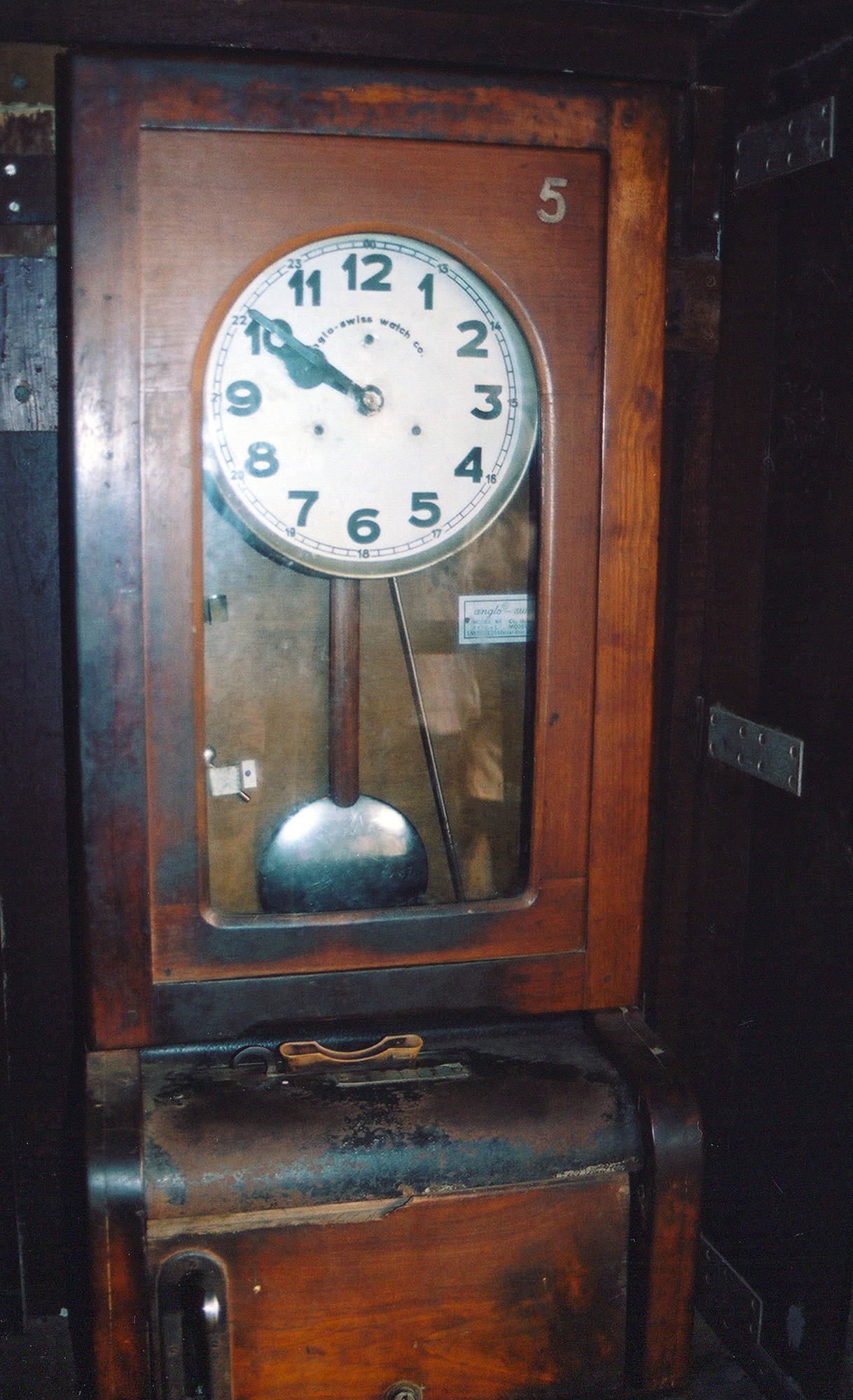This photograph captures an antique wooden clock embedded into a wooden wall. The clock is housed in a long, dark brown rectangular case, exhibiting signs of aging with darker brown weathered scuff marks all over its surface. The clock's front features a dome-arched glass cover, showcasing a white clock face with black standard numerals and hands at the top. The time displayed is 10:50. Below the clock face, a wooden rod connects to a pendulum, which has a metallic circular base. The case, which appears to have an opening mechanism though a handle is not visible, has the number 5 marked on it, along with a faint silver plaque. The background features darker wood, further emphasizing the clock's vintage charm.